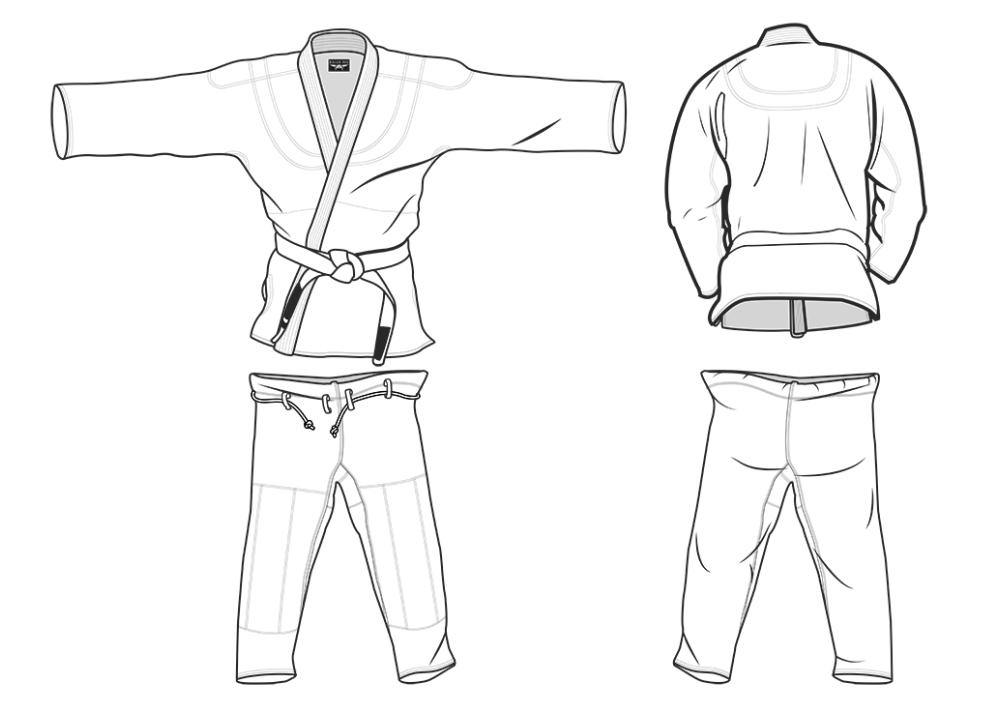The image is a detailed, black and white digital sketch of a karate uniform, arranged in a square format and divided into four sections. Each quadrant presents the front and back views of both the top and the pants. On the left, the upper left section illustrates the front of the karate jacket, which features a fold-over front with a sash tie belt knotted at the waist and long sleeves extended to each side. Below it, in the lower left section, are the matching pants with a drawstring waist, cut above the ankles. On the right side, the upper right section shows the back of the karate jacket, adorned with a gray stripe pattern across the shoulders, while the lower right section displays the back view of the pants. The entire outfit is depicted without a model, giving a clear, unobstructed view of the garment’s structure and design, possibly serving as a sewing guide. The background is white, maintaining the focus on the intricately detailed uniform.